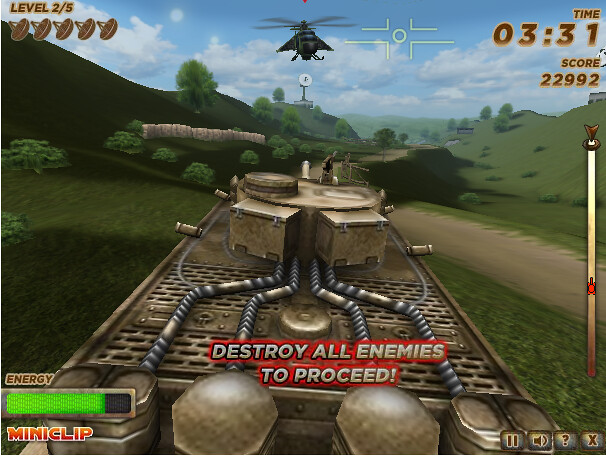The screenshot captures a dynamic scene from a video game, featuring a bright blue sky adorned with fluffy white clouds. Rolling green hills frame the landscape on both the left and right sides, dotted with sparse trees, bushes, and shrubbery. In the foreground, a large, dark gold tank with intricate piping and various equipment dominates the lower half of the image. Words on the pipes read "Destroy all enemies to proceed" against a red background. To the top right, brown text displays "Time: 03:31" and "Score: 22992". The top left corner shows "Level 2-5" with five satellite dish-shaped icons below. In the center of the screen, a black helicopter flies forward, accompanied by a reticle sight aimed nearby. A brown Humvee, armed with a gun positioned towards the helicopter, is also visible. At the bottom left, a green energy bar indicates that some energy is depleted, labeled "Energy" above. The bottom right corner includes icons for pausing the game, sound settings, a help feature, and an exit button.